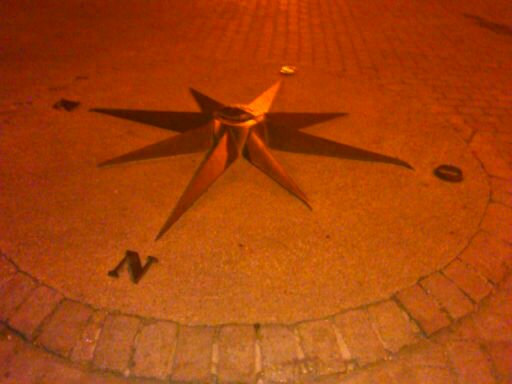The photograph captures a striking nighttime view of a large metallic compass sculpture situated in what appears to be a public courtyard, illuminated by artificial orange and yellowish lighting. The sculpture is encircled by a ring of matching bricks that seamlessly blend into the brick paths forming the courtyard. The compass features a prominently elevated circular base made of stone, decorated with ribbed trimmings along its border, and hosts an eight-pointed star at its center. Four of these points are marked with cardinal directions: ‘N’ to the bottom left, ‘E’ to the top left, ‘O’ (potentially representing 'W' for West in another language) to the right, and ‘S’ at the top. The metallic compass needles, rendered in a rich brown hue, are arranged to point towards these directions. An overhead light source casts a striped shadow, adding to the antiquated, relic-like ambiance of the setting.